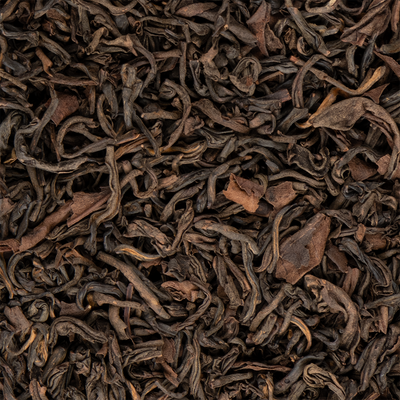This close-up photograph features a large pile of dried, brown, and occasionally green leaves scattered on the ground. The leaves exhibit a variety of shapes, with some appearing straight while others curl up into worm-like rolls, giving the illusion of dried-up worms or thin twigs. The leaves, primarily brown but with shades of green and hints of brownish-orange, cast subtle shadows across the scene, indicating their brittle and dried nature. Their textured, curled appearance adds an organic complexity to the image, portraying a detailed view of nature's process of decomposition.